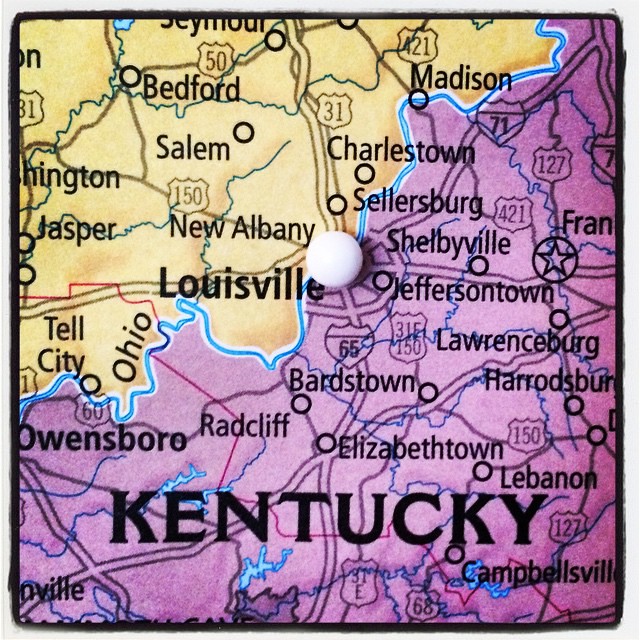This image depicts a detailed, close-up map split diagonally by a blue line, with a white pin placed at the boundary of the two sections. The top half of the map is a beigey-yellow, representing Indiana, while the bottom half is shaded in purple, denoting the state of Kentucky. The Kentucky section prominently features black lettering indicating various towns including Owensboro, Radcliffe, Bardstown, Elizabethtown, Lebanon, Harrodsburg, Lawrenceburg, Jefferson Town, Shelbyville, and Sellersburg. Positioned centrally is Louisville with the white pin marking it. In the upper left portion of the map, we see Indiana towns such as New Albany, Salem, Bedford, Jasper, Madison, Tell City, Charlestown, and Seymour. Blue waterways, including three lakes and the Ohio River, meander through the purple section of the map, outlining the geographical layout. Highways like Interstate 65 are also depicted, illustrating the connectivity across the map.